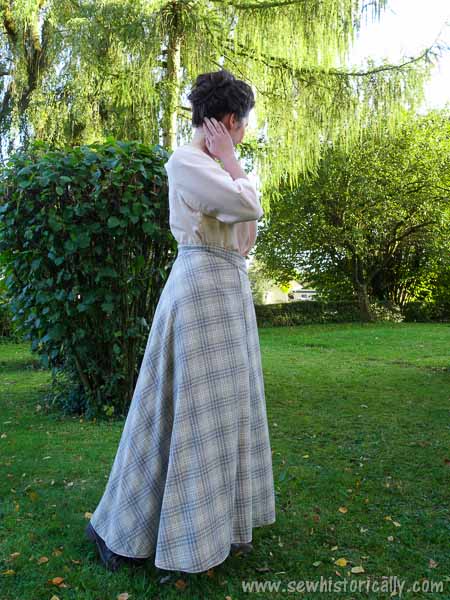The image is a detailed, close-up photograph of a woman standing in a brightly lit garden or park. She is prominently featured wearing a light pink long-sleeve shirt and a long, ankle-length skirt with a white and gray plaid pattern, which touches the ground. She stands on green grass, surrounded by lush greenery including a tall tree partially visible behind her, and green bushes both directly behind and to her right. The woman is positioned with her right arm and hand touching the back of her neck, and her dark brown hair is styled up in a bun. A watermark at the bottom of the picture reads "www.sewhistorically.com".